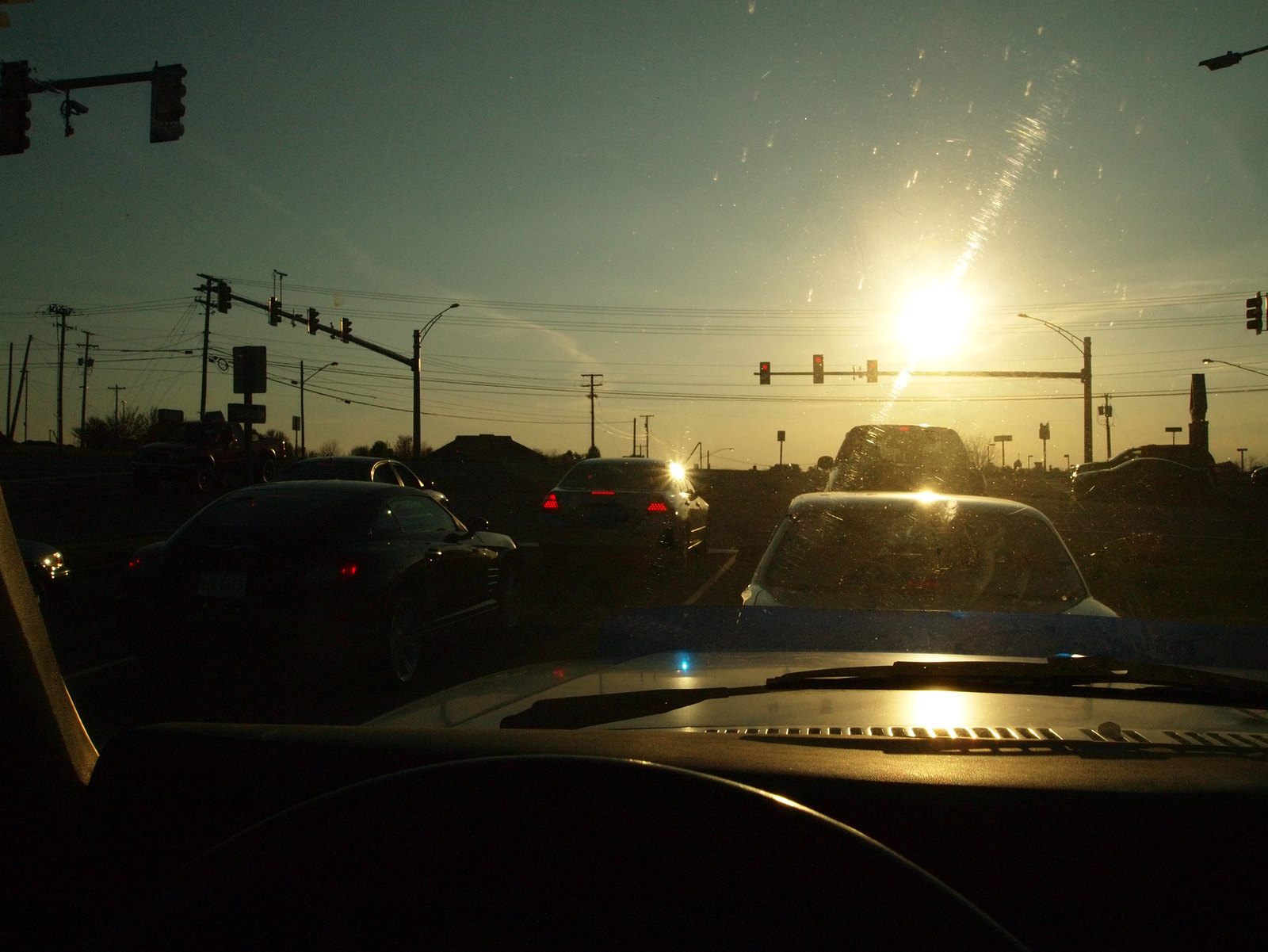This photograph captures a busy intersection during dusk, with a multitude of cars halted at a red light. The image, taken from inside a vehicle positioned in the third car on the right-hand side, offers a clear view through the windshield. Surrounding the intersection, one can observe illuminated headlights and brake lights from vehicles on the left, right, and ahead. The sky, showing signs of approaching nightfall, remains a vibrant blue with scattered clouds in the distance. Street lamps and telephone poles, totaling approximately seven, are visible along the road, some already glowing while others remain dark. The scene is accentuated by the red traffic light directly ahead, and the brake lights of vehicles in adjacent lanes, emphasizing the congestion of the moment.